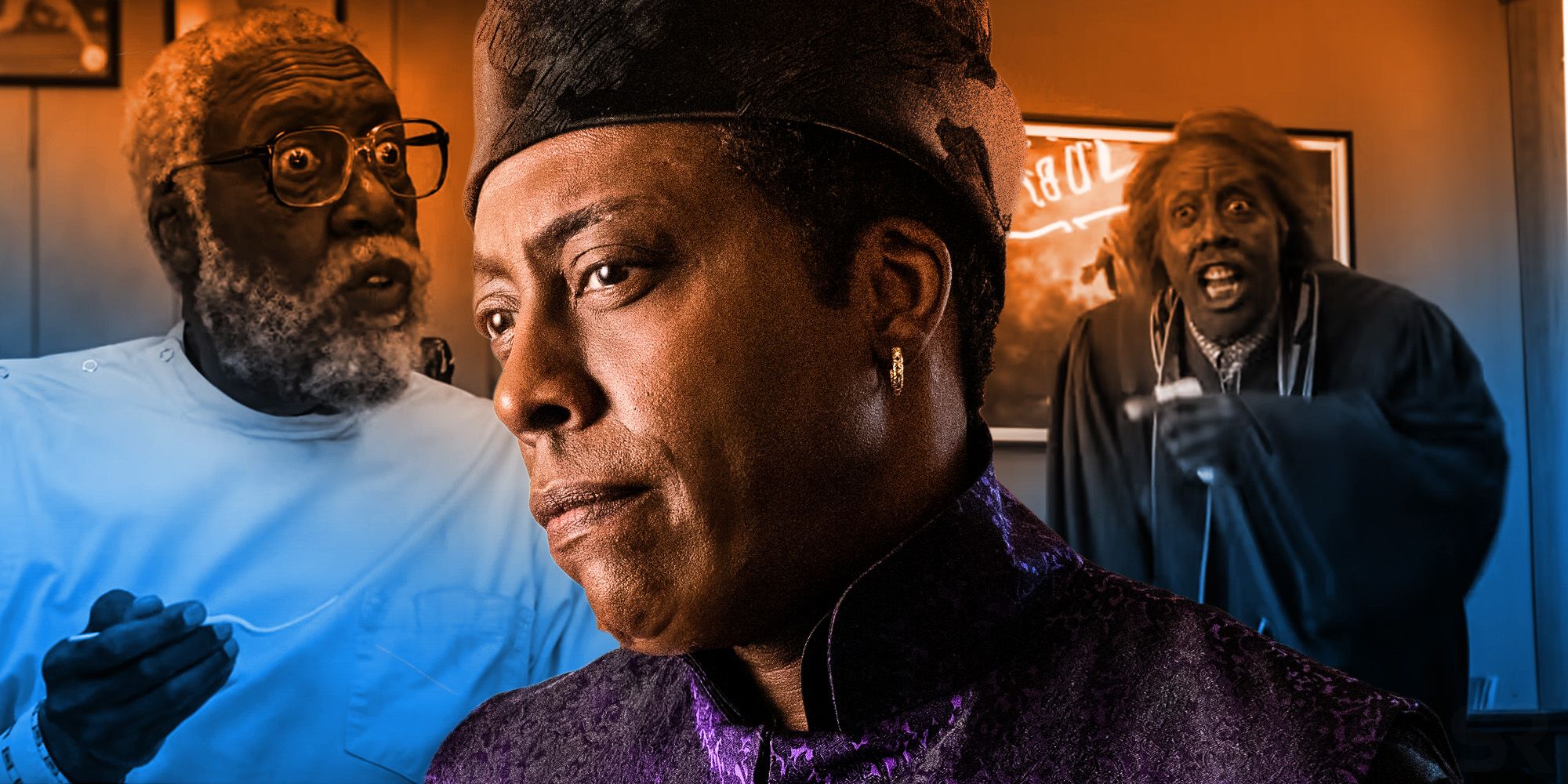In this vibrant and detailed scene from "Coming to America 2," three distinct characters, all portrayed by Arsenio Hall, are captured in a barbershop setting. In the center, Hall is dressed in a dark velvet robe with a blue-trimmed collar and wears a gold earring in his left ear along with a King Tut-inspired headdress, giving him a regal and serious demeanor. To his left, another character, also played by Hall, appears as an old black barber, clad in a blue scrub top with a white and gray beard and glasses, possibly holding a dental or barber instrument. On his right, Hall’s third character is the lively preacher dressed in flamboyant attire, echoing his wild and vibrant persona. The backdrop features an array of colors such as brown, dark purple, blue, gray, and white, enriching the barbershop's atmosphere with a warm and nostalgic feel. This captivating image showcases the versatility of Arsenio Hall, highlighting his multiple roles within a single frame.